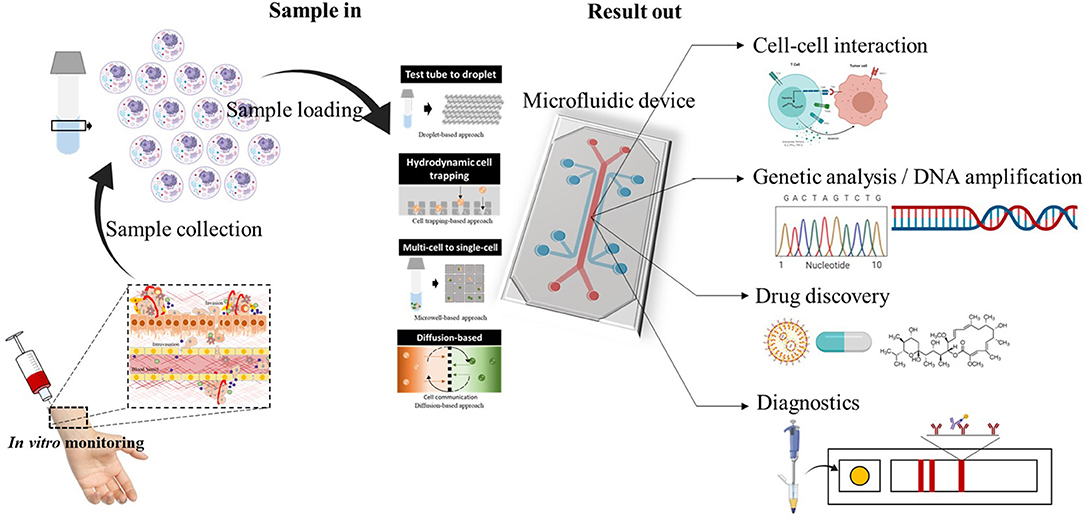This image is a detailed and comprehensive scientific diagram set against a wide white background, showcasing a medical testing procedure from sample collection to result analysis. On the left side, labeled "Sample In," there are circular biological samples and an image of a needle drawing blood from a hand, indicating the initial sample loading stage. Arrows guide the viewer through the process, illustrating sample loading techniques such as hydrodynamic cell trapping and multi-cell to single-cell diffusion-based methods.

The transition from "Sample In" to "Result Out" is indicated by a square object labeled "Microfluidic Device," which then branches into four key areas of analysis: 

1. "Cell-Cell Interaction" — depicted by an image of two interacting cells, one blue and one red.
2. "Genetic Analysis" — accompanied by visual representations of DNA and labeled "DNA Amplification."
3. "Drug Discovery" — featuring drawings of organic molecules and a pill, highlighting the potential applications in pharmaceutical research.
4. "Diagnostics" — illustrated by images of test results.

This infographic meticulously combines descriptive black text with vivid imagery to convey the step-by-step process of biological and genetic analysis within a microfluidic context for medical and research purposes.